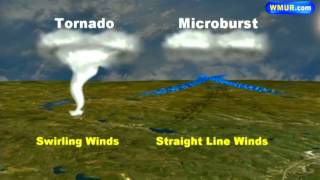This informational poster, sourced from WMUR.com, provides a graphic depiction of different dangerous weather events. The image shows a divided landscape and sky, with lush green grass, trees, bodies of water, and a cloudy, stormy sky above. On the left side of the image, a cartoon-like tornado spirals downward, labeled "Tornado" with the description "Swirling Winds" written in yellow underneath. The right side illustrates a microburst, with white clouds at the top labeled "Microburst." Blue lines extend downward and outward from these clouds, depicting the crisscrossing forces of wind, and the term "Straight Line Winds" is written in yellow below. The visual effectively contrasts the specific wind patterns associated with tornadoes and microbursts.